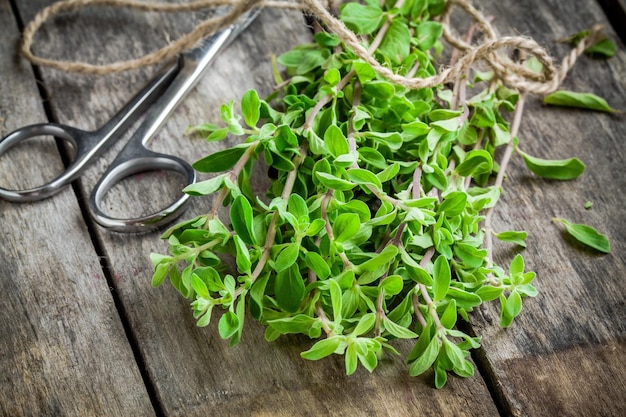The image showcases a rustic wooden table, possibly made from an assortment of weathered plywood strips, featuring hues of light tan, light to dark gray, and occasional black streaks. Resting on the table, towards the left, is a pair of small, surgical-like stainless steel scissors. Adjacent to the scissors is a bunch of vibrant green leaves, possibly herbs like parsley, with light tannish-brown stems. Draped over both the scissors and the leaves is a thick, brown yarn-like rope, loosely looped. The items appear to be part of a project involving the preparation of herbs.